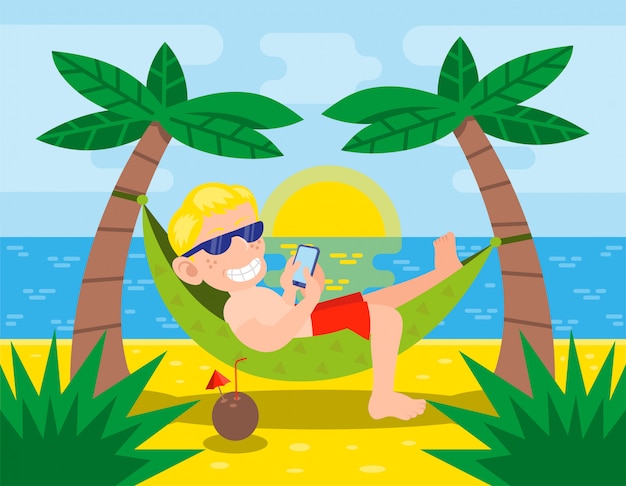In this whimsical cartoon illustration, a man with blonde hair and blue sunglasses lounges in a lime green hammock adorned with triangle designs. The hammock is attached to two palm trees, creating a relaxed beach scene. The man, wearing red swim trunks, has his right foot touching the sandy ground while the rest of his body reclines comfortably in the hammock. He holds a cell phone and turns toward the viewer with a broad, cheerful smile. Next to the hammock on the yellow and white-spotted sand rests a coconut drink with a red straw and a small red umbrella. A green bush sits in the foreground, while the background features a serene blue ocean dotted with white, gently reflecting the yellow hues of the sun. The light blue sky is scattered with white clouds, completing the idyllic vacation setting.